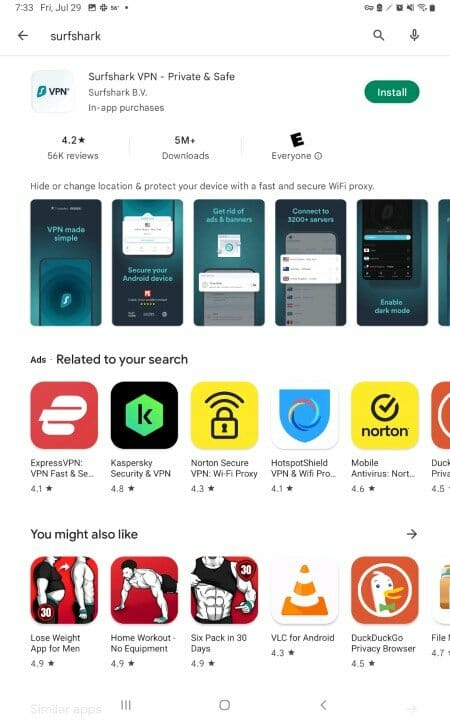A detailed caption for the given image might be:

"This is a screenshot from a mobile phone showcasing the Surfshark VPN app in an app store. At the top of the screen is a search bar with the text 'Surfshark' typed in. The background of the app store is white, while the text is in black. In the upper left corner, an icon featuring a square with the letters 'VPN' in the center is visible. Adjacent to the icon is the app’s title, 'Surfshark VPN – Private & Safe,' followed by the developer's name, 'Surfshark BV,' and a note indicating 'In-app purchases.' To the right is a green oval button with 'Install' written in white letters. Below this section, the app’s rating is displayed as '4.2 stars,' alongside text that states it has '5 million+ downloads' and is rated 'E for Everyone.' The screenshot also includes five preview images of the app, each featuring a predominantly blue-green gradient. Additionally, there are two sections displaying other apps: 'Related to your search' and 'You might also like.'"